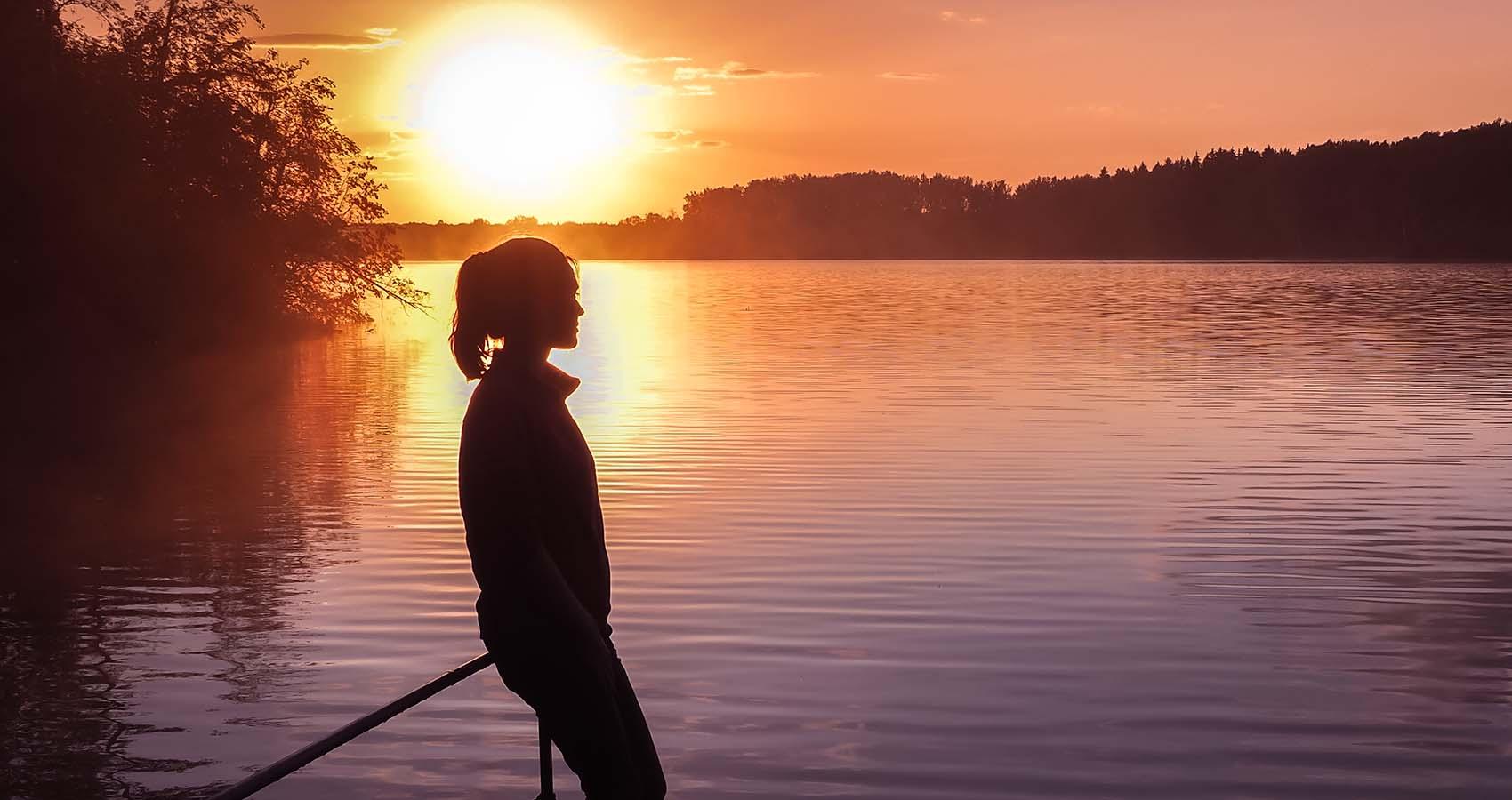The image depicts a woman standing on a dock or pier along the edge of a calm, large-bodied lake. With her hands tucked into the pockets of her fleece, she leans casually against a railing, her long, somewhat messy hair tied in a loose ponytail. The scene is bathed in the warm, hazy glow of either sunrise or sunset, as the sun, partially obscured by the horizon, casts an orange and yellow hue across the sky. The sunlight creates a striking silhouette of the woman, highlighting her contemplative stance. In the background, a dense forest frames the horizon, and a single bushy tree tilts into view from the left side of the image. Scattered clouds and a slight mist hover over the serene water, which gently mirrors the soft light of the setting (or rising) sun.